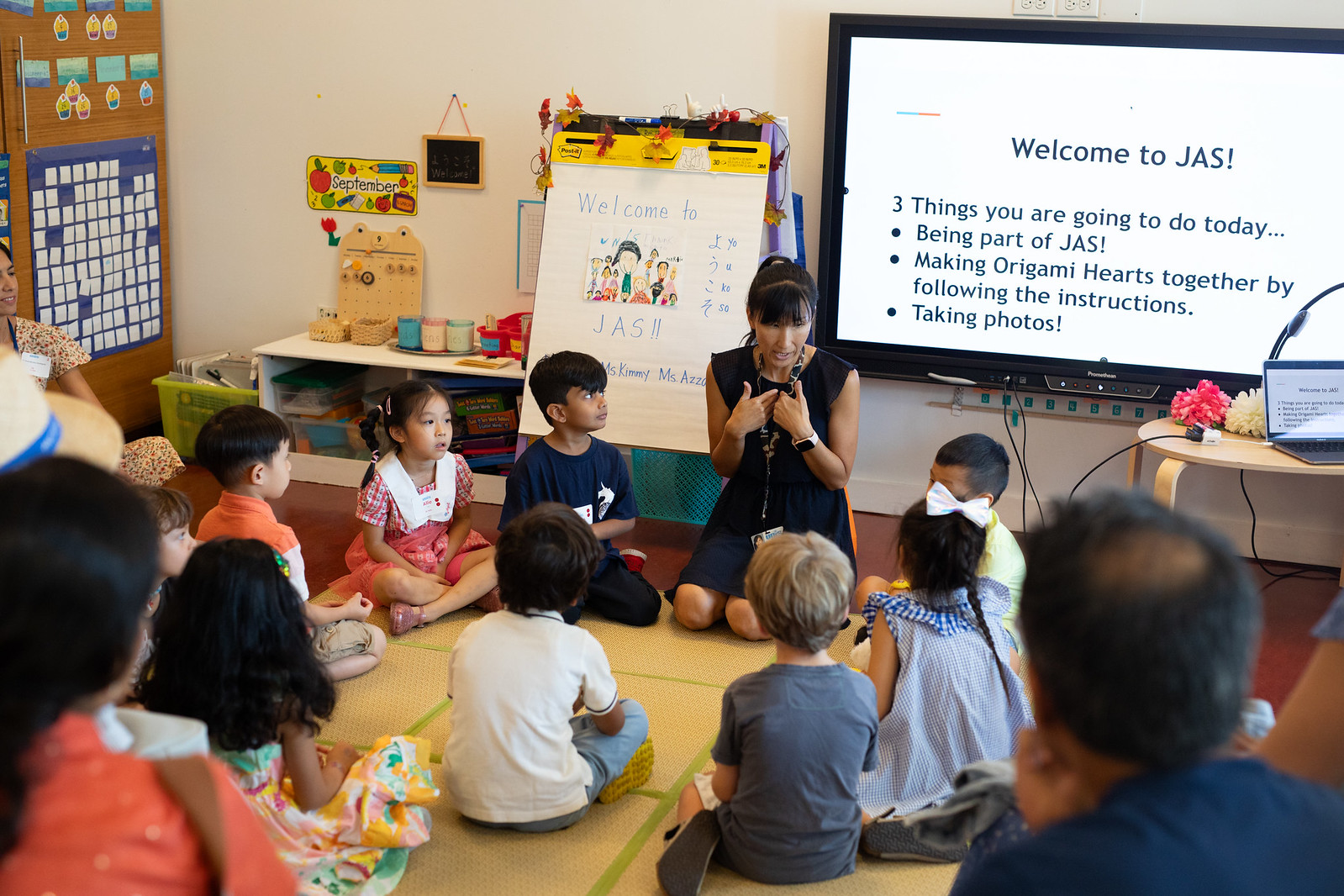In this vibrant classroom scene, a group of nine or ten children, who appear to be Asian, are sitting cross-legged on a colorful yellow and green mat, forming a circle around their teacher. The teacher, dressed in a blue dress with dark hair, is seated on her knees and intently engaging with the children. Her attention is directed downward as she speaks to them. 

Behind the group, there is a prominent white screen displaying in black text, "Welcome to JAS." The screen details three activities for the day: making origami hearts by following instructions, talking, and taking photos. Below the screen, a visible power strip and cords suggest a connected setup in the room.

On the right side of the image, in front of the screen, stands a round table with an open laptop, accompanied by two flower displays, adding a touch of nature to the indoor setting. Adjacent to the teacher on her left is a chart with paper, reading "Welcome to JAS," likely detailing the day's agenda or classroom rules.

The children, intently listening to the teacher, include a little boy in a blue shirt, a girl with a white-collared dress seated next to him, and another boy in an orange shirt. The background reveals white walls adorned with various educational posters and charts, including a board labeled "September" and a smaller chalkboard.

On the far left, there is a shelf stocked with colorful paints, toys, and puzzles, indicating a well-equipped learning space. Additionally, partial views of some parents in the background suggest they are observing the session. The overall atmosphere is one of focused, engaged learning, filled with colorful and organized educational tools.